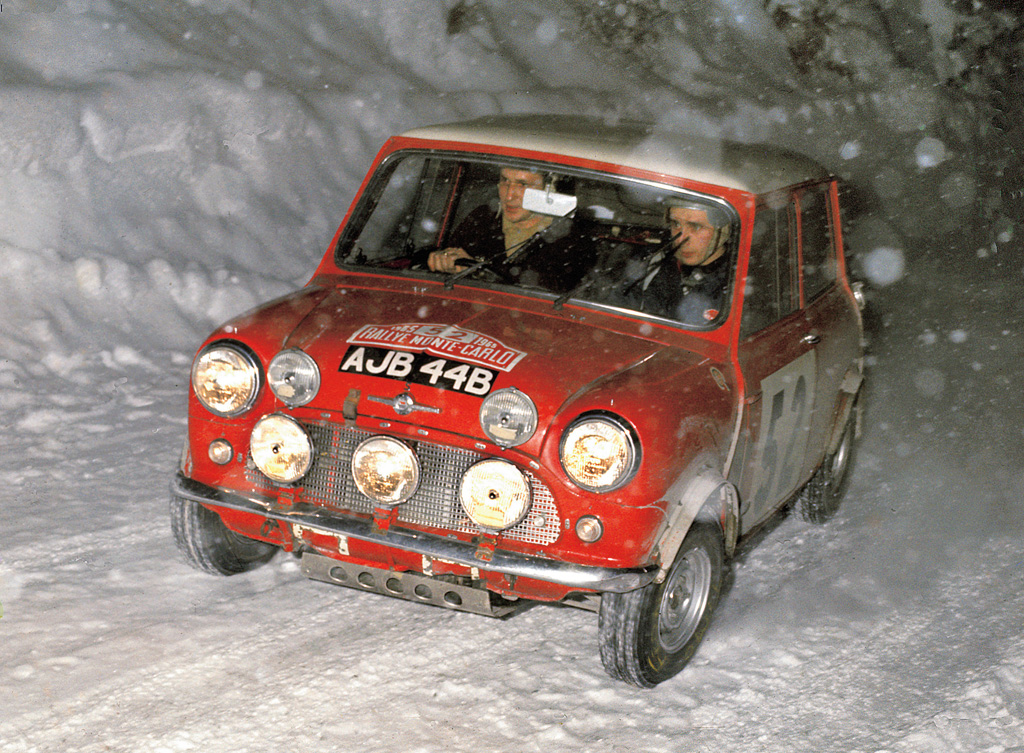The image depicts a vintage, small, red car, reminiscent of a Mini Cooper or an old sedan from the 1970s or 1980s, racing through a snowy landscape. The car features multiple circular rally lights on its grille, specifically five at the front and two on the fenders. It has a white roof and is adorned with the insignia "Rally Monte Carlo 1958" on the hood and the number "52" in black text on a white background on the right-hand side door. Additionally, the tag number "AJB44B" is also present on the vehicle. The red car, driving on a snow-covered, plowed road with visible tire tracks, is right-hand drive and occupied by two individuals. The driver is on the right, with a focused expression, and the navigator on the left. Both appear to be wearing black jackets, possibly uniforms, and helmets. A large snowbank looms behind them, while snow continues to fall in the backdrop, indicating a harsh winter environment. Trees are visible in the upper right corner of the image, and the overall scene captures an intense moment during a nighttime rally event.